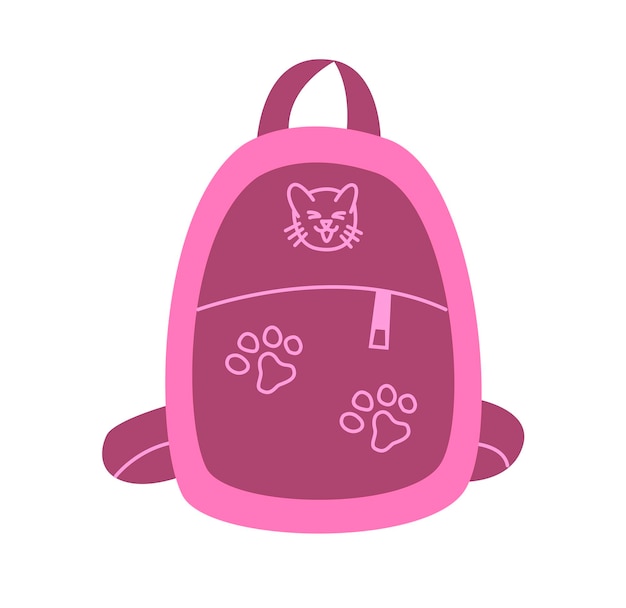This illustration depicts a child's backpack centered within a square frame. The backpack, primarily pink, features a dark purple center shaped like an Easter egg. A smiling cat face, also outlined in pink, adorns this dark purple section, with three whiskers on each side, two ears, and two eyes. Below the cat face, there are two pink-outlined paw prints within the purple area. A horizontal zipper, with a pink pull tab designed as a dangling rectangle with a square cut out, runs across the dark purple center. The top of the backpack has a dark purple strap, shaped like an upside-down U, matching the central section's color. The backpack also has visible straps, one at the very top and two on either lower side, blending shades of pink and burgundy.